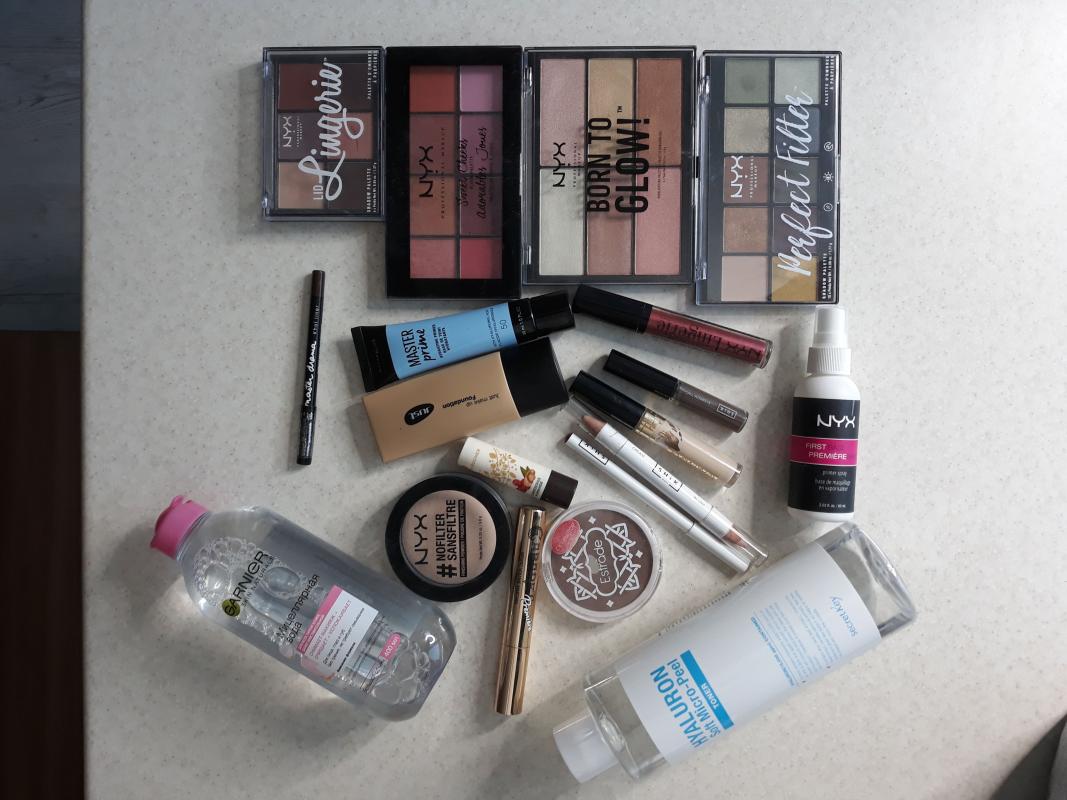This photo showcases a well-organized marble vanity counter, primarily white in color with subtle grayish speckles. At the top of the counter, neatly aligned, are several makeup palettes: a six-color eyeshadow palette, an eight-color eyeshadow palette, and a six-color lip gloss palette, alongside a ten-color eyeshadow palette. At the bottom of the image, there is a bottle of Garnier Micellar Cleansing Water. On the opposite side, there is a clear bottle with a white label containing hyaluronic micro peel. The space between these items is filled with various beauty products, including a spray bottle, a small tube of primer, foundation base makeup, eye pencils, lip pencils, concealer, lipstick, eyeliner, and mascara. The entire arrangement exudes a sense of meticulous organization and readiness for a detailed makeup routine.